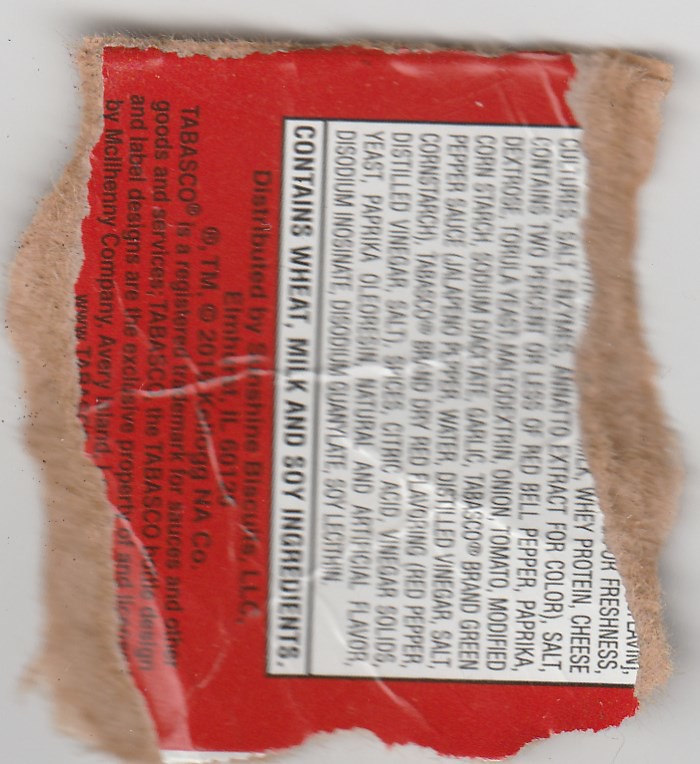The image, slightly rectangular in a vertical orientation, features a somewhat blurry depiction of a torn section of box packaging against an off-white background. The ripped packaging is central to the frame and displayed sideways, with the bottom of the label oriented to the left and the top to the right. The torn edges reveal light tan cardboard on both the right and left sides. In the center, there is a red label background that includes the lower portion of a white nutritional facts box, adding a touch of contrast to the overall scene.